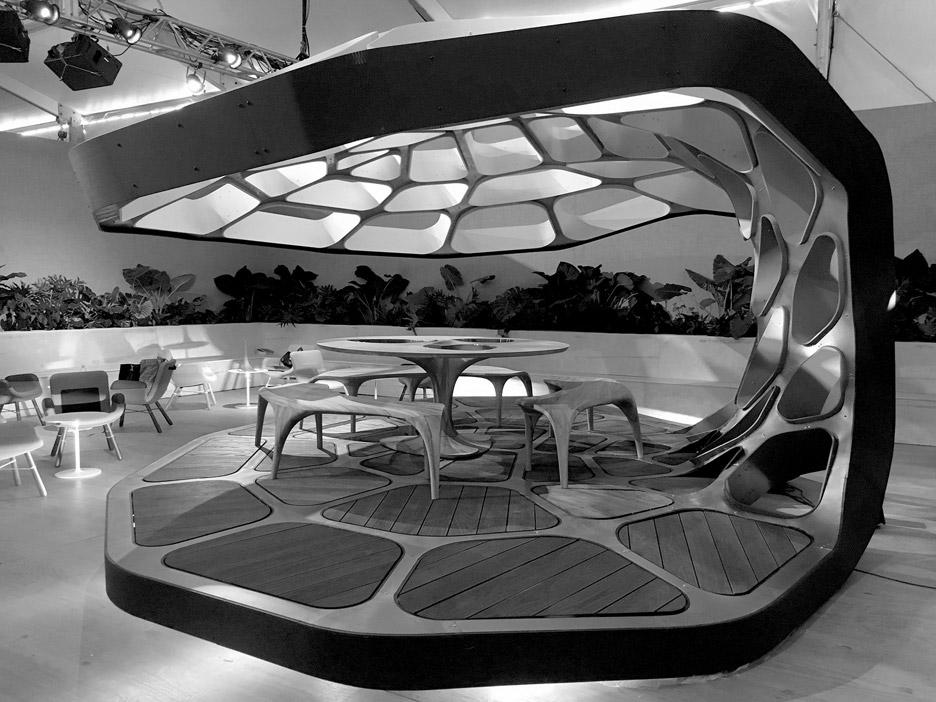This black and white photograph showcases a strikingly futuristic, mid-century modern stage or movie set bathed in professional studio lighting. The central feature is a unique C-shaped platform with a honeycomb-like structure of wooden plates, which extends upwards to create an overhang. This honeycomb is punctuated with open holes, allowing light to filter through from above. At the core of this elevated platform stands a circular table surrounded by three curved benches, echoing the modernist design aesthetics of the 1960s space-age furniture.

Encircling this central arrangement, the room is furnished with several mid-century modern café tables accompanied by armchairs with ring backs. The perimeter is adorned with planters brimming with broad-leafed indoor plants, contributing to the room’s lush atmosphere. Above, a network of lighting rigs and beams supports multiple professional lighting rings, ensuring the set is well-illuminated. This meticulously crafted space exudes an air of abstract functionality, blending artistic geometric forms with practical seating arrangements, making it resemble a futuristic cafeteria or a potential eclectic art installation.